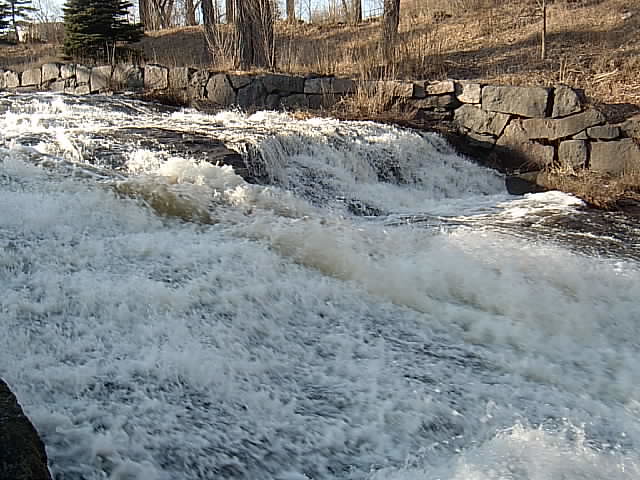A turbulent, rushing river cascades down several levels, creating a series of mini waterfalls with frothy white water splashing vigorously over rocks. The water is swift and rough, especially in the center where it appears almost pure white against the brown rocks underneath. The river is bordered by a flat rock wall, gray in color, which lines the banks and forms a barrier. Above the rocks, a hillside of brown earth and dead weeds rises, punctuated by a few leafless tree trunks. In the upper right corner, only the barren hill is visible, while the upper left is framed by two green evergreen trees. Behind the hillside, there's a glimpse of light blue sky peeking through the tall, sparse trees. The overall scene is a dynamic and rugged slice of nature, filled with the colors of white, green, brown, and gray.